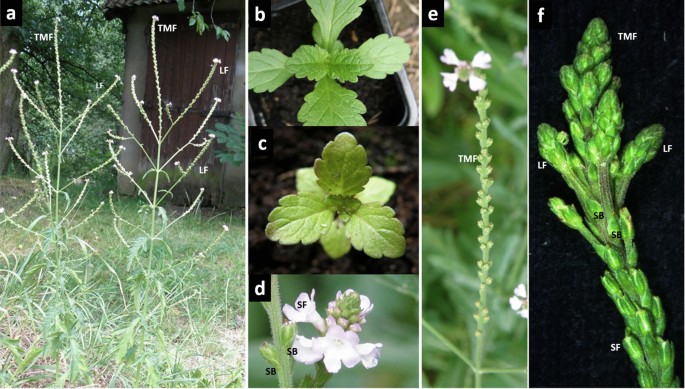The image is a detailed botanical diagram showcasing a specific plant, meticulously labeled from A to F. The first photograph (A) illustrates the full plant with a tall, spindly structure typical of flowering weeds, visibly set against a background that includes an old barn door. The subsequent images B, C, and D provide close-up views focusing on various aspects of the plant. B highlights the stem base, with notched protrusions, while C and D offer top-down perspectives of the veined leaves branching in clusters of three or four. Image D further reveals a delicate cluster of purple flowers resembling snapdragons. Image E provides a zoomed-out perspective of the flowering stalk, likely the same as that captured in D but without visible flowers. Finally, image F showcases tightly closed, grayish flower buds resembling asparagus heads, suggesting an early stage of the budding process seen in images D and E. Each photograph is notated with specific letters or numbers to indicate and describe individual parts and features of the plant in great detail.